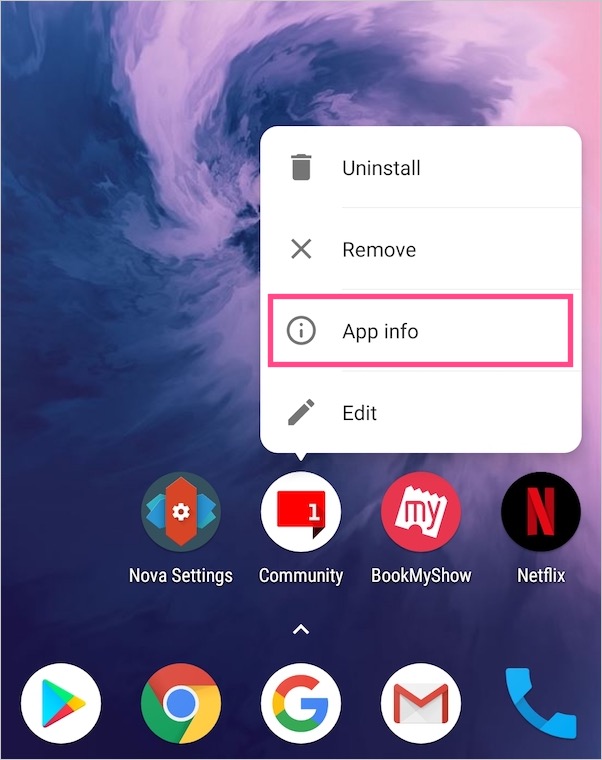The image depicts the home screen of a smartphone with a visually striking background that resembles a whirlpool. At the bottom of the screen, the dock contains several commonly used apps. From left to right, these are the Google Play Store, Google Chrome, the Google app, Gmail, and the Phone app. Above the dock, the screen displays various apps including "Nova Settings," "Community," "Book My Show," and "Netflix." The "Community" app is currently selected, and an action dialogue box is open with the options to "Uninstall," "Remove," "App Info," and "Edit." The "App Info" option is highlighted in pink.